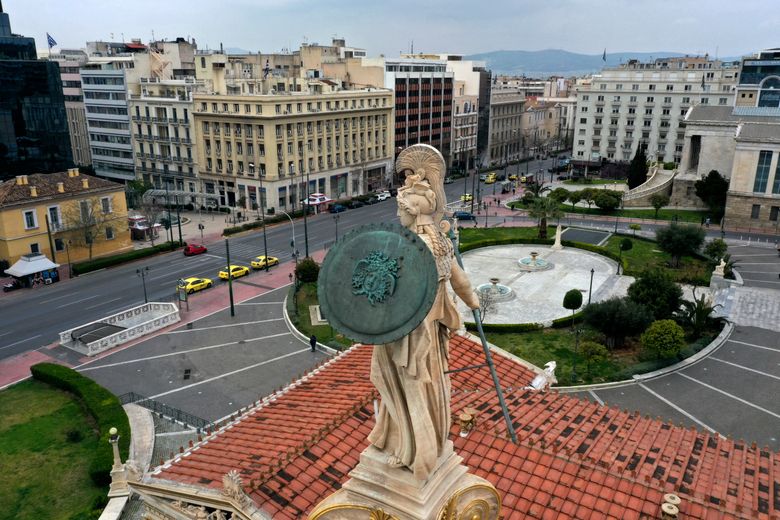The image captures a high-angle view of an urban landscape dominated by a majestic statue of the Greek goddess Athena. The statue, made of an ivory-colored material, stands proudly atop a tall white pedestal adorned with gold decorations, positioned on a red-tiled roof. Athena is depicted wearing flowing robes and a tall crested helmet, holding a large bronze shield emblazoned with Medusa's head, and a spear, both corroded to a green patina.

Beneath the statue, the roof displays patches where tiles are missing, revealing black spots. Surrounding the base of the structure, there's an open area with bushes, trees, and grass, resembling a small garden. Below the roof, there's a parking lot with visible cars, and nearby streets bustling with additional vehicles, including taxi cabs. The scene extends into a vibrant cityscape, filled with more buildings and streets, while the far horizon is framed by distant mountains, adding a picturesque backdrop to the city.